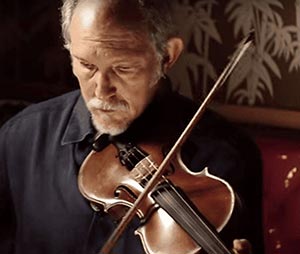The image depicts an old man with balding white hair, a white mustache, and a bit of white stubble on his chin, wearing a black collared shirt. He is holding a dark brown wooden violin under his chin, seemingly preparing to play it as he looks down towards the bottom left, possibly at a piece of sheet music. His right hand, holding the violin, is visible in the lower right corner of the image, while the hand holding the bow is not fully visible. The bow rests across the middle two strings of the violin. The setting appears to be an interior room with a red lower wall and a dark brown upper wall adorned with white plant-like designs. The photo has a grainy, low-resolution quality, possibly due to being a still from a video or a heavily cropped and enlarged image.